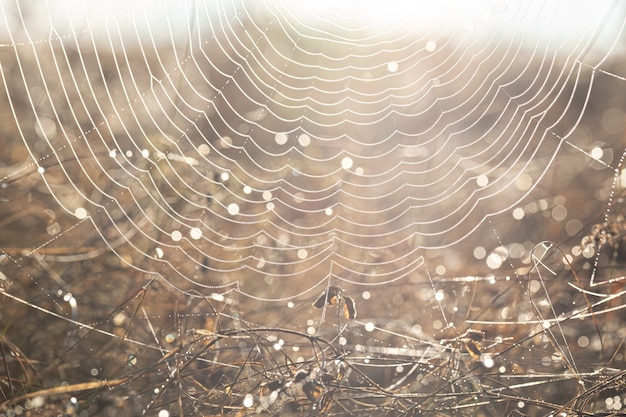This is a close-up photograph of an intricate spider web near the ground, attached to various twigs, pieces of grass, and other bits of plant life. The web's strands form concentric and wavy patterns, stretching out in multiple directions. Water droplets cling to the web, reflecting light and creating tiny, out-of-focus spots throughout the image. The background is slightly blurred, emphasizing the delicate structure of the web. The photograph is backlit, with strong light, likely from the rising sun, washing out the top portion and casting a bright glow across the scene. The interplay of light and moisture gives a subtle shimmer to the spider web, highlighting its complex beauty against the earthy backdrop.